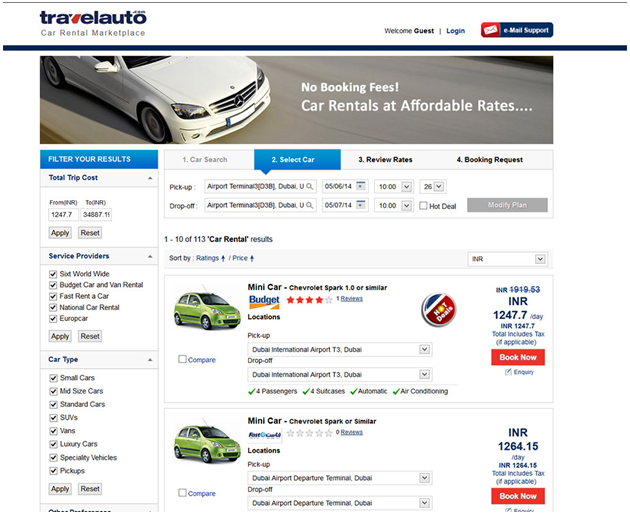This image captures a detailed desktop screenshot of a car rental website, designed to facilitate the booking of rental cars for travel. At the top left corner, there is a header titled "Travel Auto Car Rental Place," under which it greets users with "Welcome Guests" and offers options to "Login" or obtain "Mail Support."

Dominating the center of the screen is a prominent picture of a white car, accompanied by promotional text highlighting "No Booking Fees" and "Car Rentals at Affordable Prices." To the left side of the screen, users are provided with various filters to refine their search. The filters include options to sort results based on total trip costs, which appear to be displayed in Indian Rupees (INR) ranging from ₹1,247.70 to ₹34,887.15. There are buttons to "Apply" or "Reset" these filters.

Service providers can be chosen from a list that includes Sixt Worldwide, Budget Car and Van Rental, Fast Rent a Car, National Car Rental, and Europcar, with options to "Apply" or "Reset" preferences. Below these filters are categories for car types, such as Small Cars, Midsize Cars, Standard Cars, SUVs, Vans, Luxury Cars, Specialty Vehicles, and Pickups.

Further down, although partially obscured, another set of filters or settings seems to be present. To the right, a series of tabs guide the user through the booking process: "Car Search," "Select Car," "Review Rates," and "Booking Request." Users can specify the pickup and drop-off locations and dates, which in this case suggests the rental period is just for one day.

Two car options are displayed for selection. The first option is a "Mini Car, Chevrolet Spark 1.0 or similar," rated four stars and available for pickup and drop-off at the Dubai Airport. This vehicle accommodates four passengers and four suitcases and includes features like automatic transmission and air conditioning. It's advertised as a "Hot Deal," with the original cost listed as ₹1,919.63, but discounted to ₹1,247.70 per day, inclusive of any applicable taxes, with a "Book Now" option.

The second car listed is identical in model and features but is offered by a different provider, Fast Rent a Car, at a slightly higher rate of ₹1,264.15.

In essence, the screenshot provides a comprehensive overview of the car rental booking interface, highlighting the process and options available for users seeking rental cars.